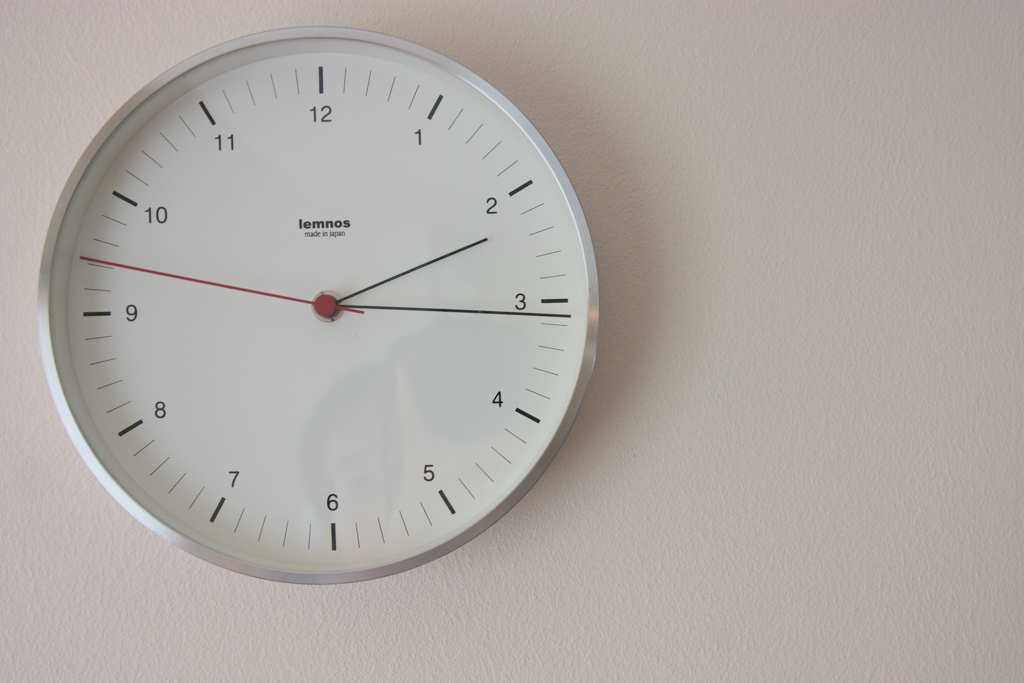The photograph features a clock situated against a textured white wall, positioned on the left side of the frame rather than centered. The clock boasts a sleek metallic silver casing around a pristine white face. Its minimalistic design includes narrow black hour and minute hands, accompanied by a long, striking red second hand. The hours are denoted by clear numerals, with additional hatch marks in between each numeral to indicate every 12 minutes. At the top center of the clock face, the brand name "lemnos" is inscribed in lowercase black font. Just below the brand name, the phrase "made in japan" is subtly printed in a smaller black font, adding to the clock's understated elegance.